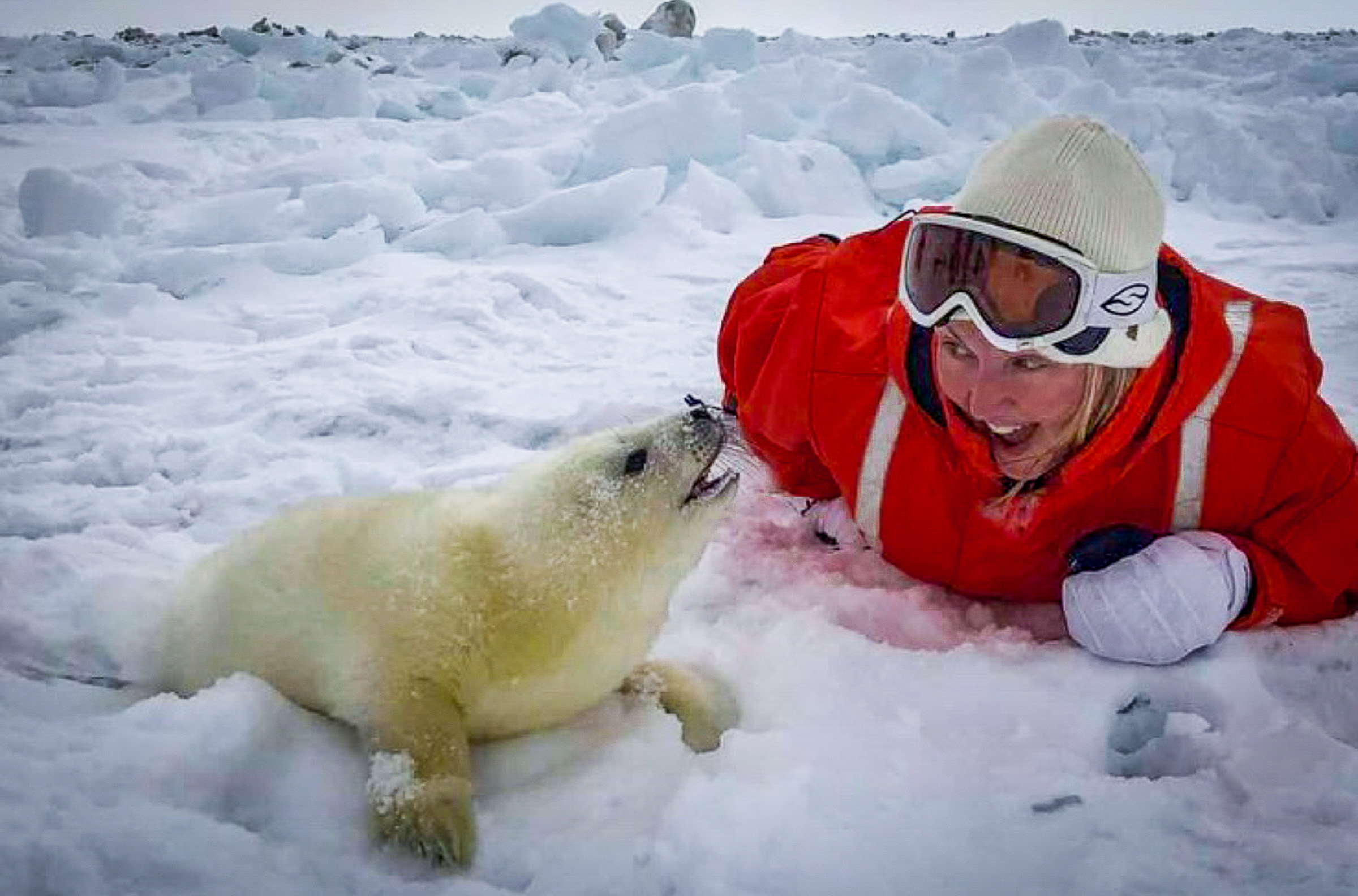In a horizontally aligned rectangular image set amidst a vast, snowy landscape in what appears to be the Arctic Circle, a woman dressed warmly lies on her stomach in the snow. She is wearing a thick red coat with white accents, white mittens, and a white beanie with ski goggles pushed up onto her forehead, revealing her blonde hair beneath. The woman is grinning widely, her mouth open, as she engages with a baby seal to her left. The seal, covered in fluffy white fur and speckled with tan spots, lies with its head tilted upwards, mouth open as if making a sound, appearing almost to smile back. The snow beneath the woman has a slight pinkish hue, and behind them both, clumps of icy snow pile up against a backdrop of gray sky. The scene exudes a moment of joy and connection between the woman and the curious young seal, capturing an intimate wildlife encounter in the midst of a frozen wilderness.